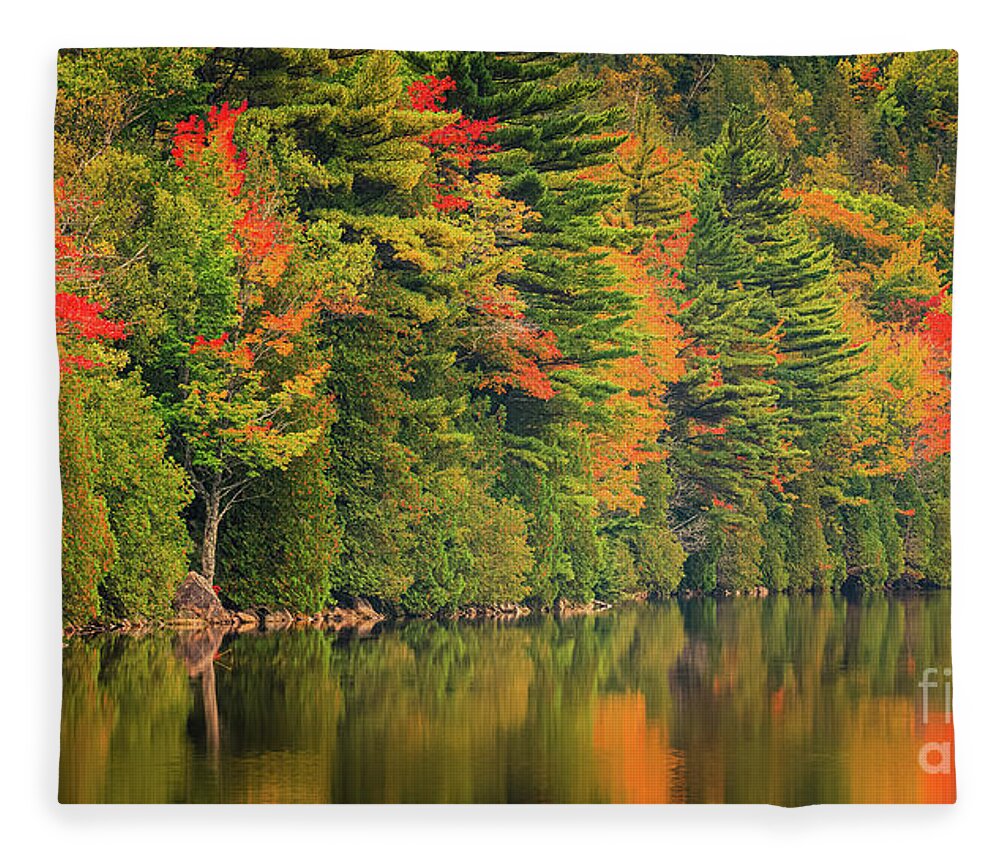This detailed nature photograph captures the serene edge of a river or lake, surrounded by a dense and tall forest of striking beauty. The scene features a multitude of trees including green pines, as well as deciduous trees with leaves in brilliant fall colors—red, orange, and yellow—indicating the season is autumn. The water is remarkably clear and reflective, mirroring the stunning array of colors from the trees above, though the reflection appears somewhat blurry. On the left side of the image, a large rock is positioned in front of one of the trees. The photograph has some writing in the lower right-hand corner that appears to be cut off, suggesting it might be part of a larger image or some form of advertisement.